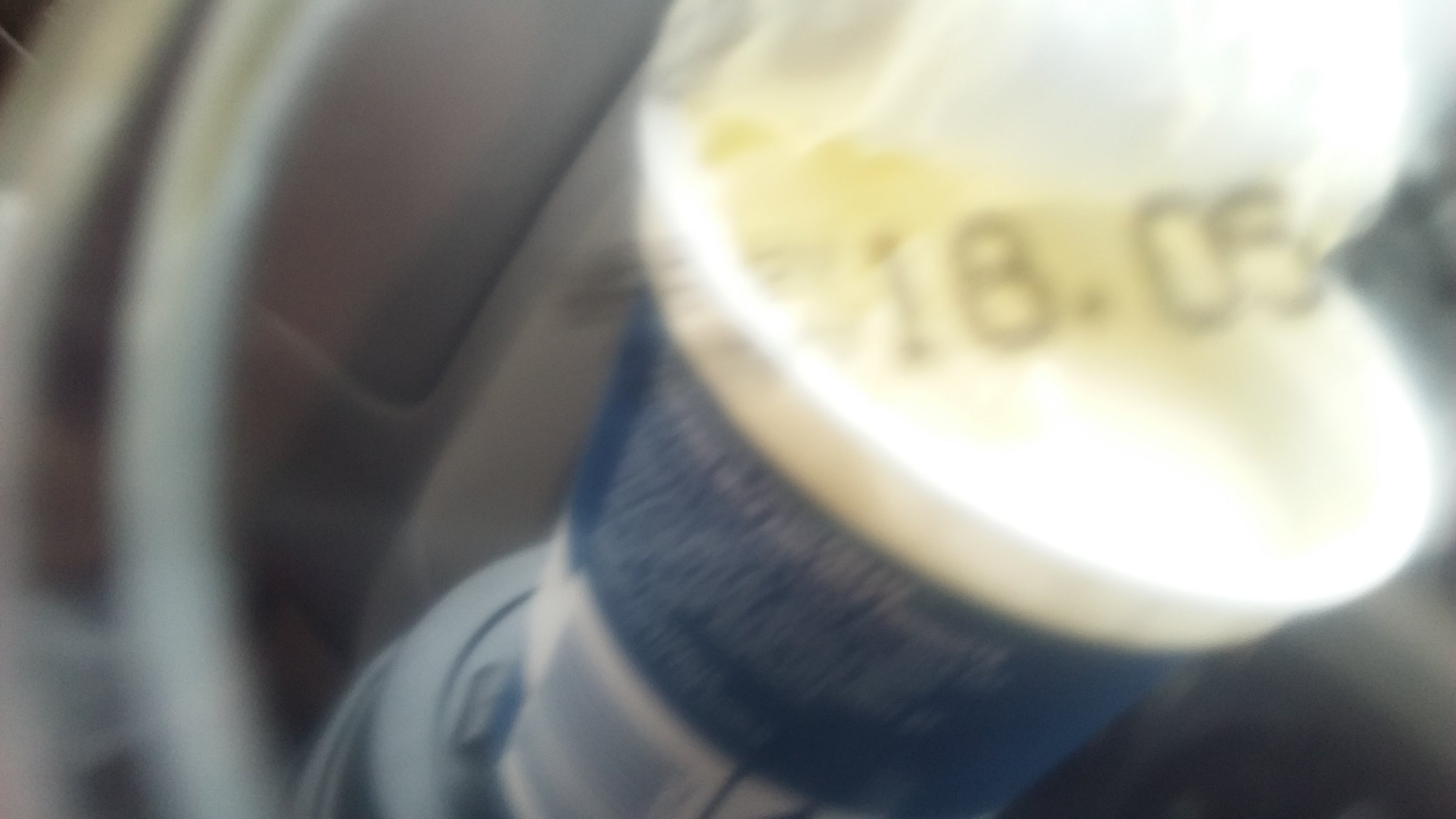The photograph captures a blurry, mid-motion close-up of a plastic container with a matching lid, most likely designed for holding food or beverages. The container appears to be filled with a thick, white, creamy substance, though the exact nature of the contents is unclear—it could range from a dairy product to a type of paint, given the lack of fine details. This container is situated on top of a coffee cup holder within the interior of a car. A date stamp is visible on the container, but it is illegible due to the blurriness and poor focus of the image.